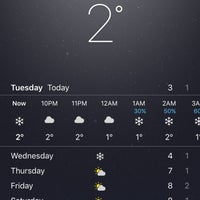This image is a screenshot of a weather application on a mobile phone. The app displays information based on the user's current location and is shown in a dark theme, indicative of nighttime. In the center, the temperature is prominently displayed as 2°C. The date is marked as Tuesday, and the current time is indicated as 10 PM.

The hourly forecast starts with a "now" section featuring a snow icon and a temperature of 2°C. Following this, the weather forecast for 10 PM and 11 PM both show a cloud icon with a temperature of 2°C. For 12 AM, the cloud icon persists, but the temperature drops slightly to 1°C. This pattern continues with a breakdown of the forecast into subsequent time slots: 

- 3 AM: Snow icon, 1°C.
- The forecast continues intermittently throughout the night into the morning.

Towards the bottom of the image, the forecast extends into the upcoming days with labels for Wednesday, Thursday, and Friday. The temperatures for these days are listed on the right-hand side, showing a progression of numbers: 4°C, 7°C, 8°C, followed by a series of 1°C markers and concluding with 2°C. 

Overall, the image provides a detailed and comprehensive hourly breakdown of the weather conditions, emphasizing cloud cover and potential snowfall throughout the night into the early morning hours, with an extended forecast for the upcoming days.